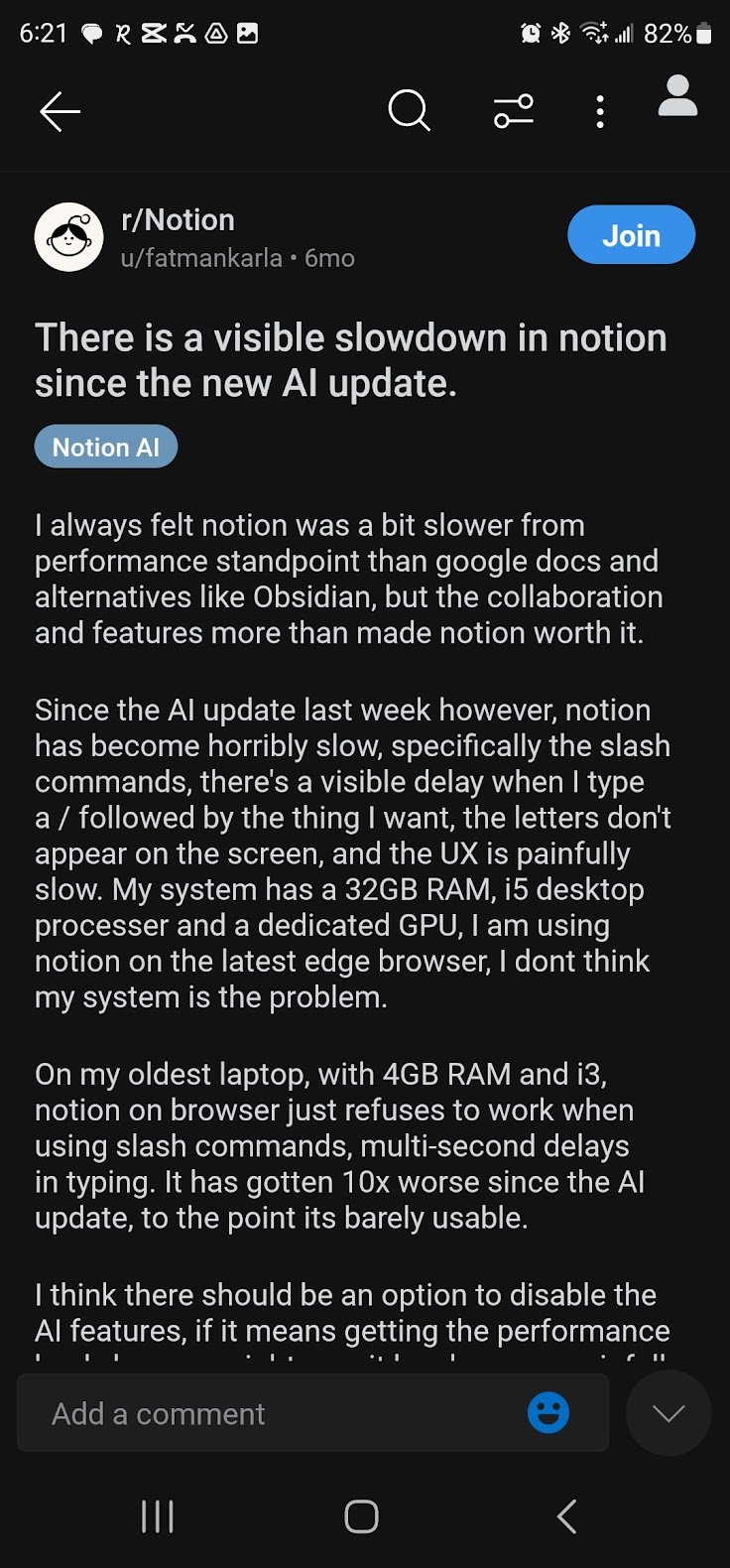This detailed screenshot depicts a Reddit response from the r/Notion subreddit, focusing on the performance issues in Notion following a new AI update. At the top of the image, there's a noticeable headline stating concerns about a slowdown in Notion since the AI update, labeled with the tag "Notion AI."

The post contains three fully-visible paragraphs and a partially-visible fourth paragraph. The author begins by comparing Notion's performance unfavorably to Google Docs and Obsidian, noting that while Notion's collaboration features previously compensated for its slower speed, the latest AI update has drastically worsened the user experience. They specifically highlight a significant delay when using slash commands, where the letters fail to appear on the screen promptly, making the user experience excruciatingly slow.

The author mentions their hardware setup—a system with 32GB of RAM, an i5 desktop processor, and a dedicated GPU—running Notion on the latest Edge browser. Given this configuration, they express doubt that their system is at fault. They further illustrate the problem by describing their experience on an older laptop with 4GB of RAM and an i3 processor, where Notion in the browser becomes unusable with multi-second delays in typing, worsening considerably since the AI update. 

The post concludes with a strong suggestion for an option to disable AI features to regain lost performance. Unfortunately, part of this final paragraph remains partially visible in the screenshot.